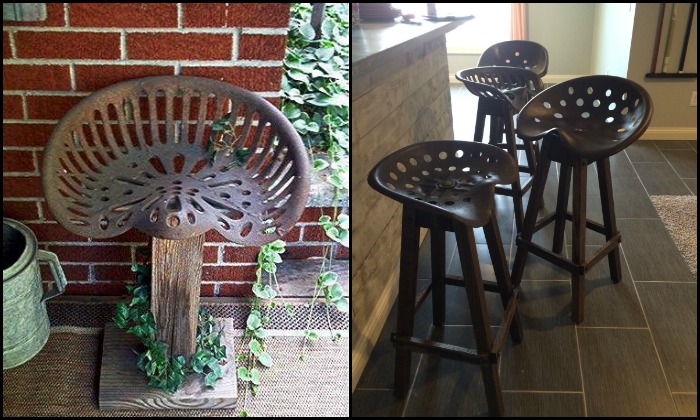The combined image consists of two separate photos, each bordered by a thin black line. The left photo features a rustic scene with a wooden pedestal topped by a metallic tractor seat that has been artistically transformed, featuring intricate holes and a slight backrest. This structure stands against a red brick wall. Green vines wrap around the seat and extend towards the right, growing along the wall. To the left of the seat, a silver bucket can be seen. The right photo showcases a kitchen setting with three brown bar stools, also fashioned from repurposed tractor seats with similar hole patterns. These stools are positioned on a dark grayish-brown tiled floor and are placed beside a counter.